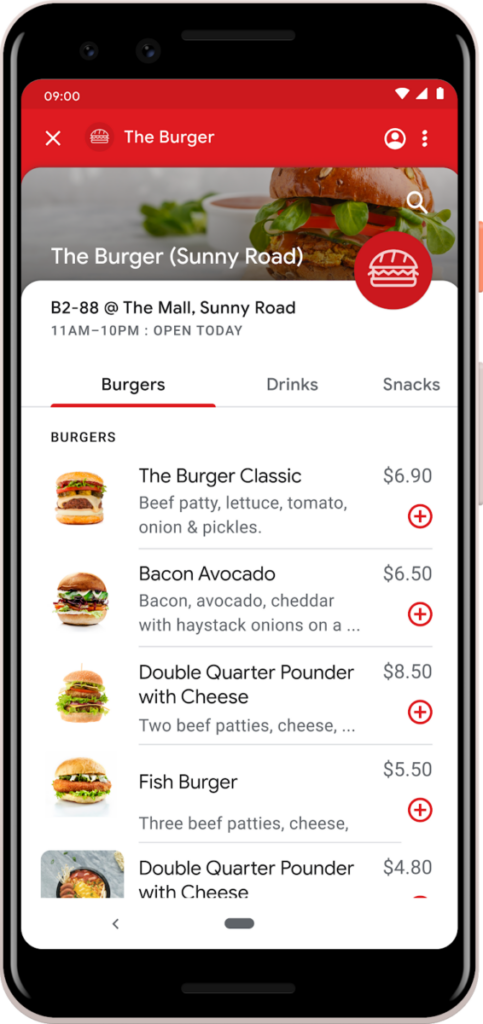A screenshot of a phone display features a detailed promotional banner for a burger restaurant. At the top, a red banner displays the current time as 9:00 AM along with a fully charged battery icon. The banner includes a left-aligned 'X' button, a hamburger menu icon labeled "The Burger," and three vertical dots on the right for additional options. Below the banner, the restaurant name "The Burger" is reiterated, with the location "Sunny Road" in parentheses next to it.

The background image features a delicious hamburger topped with fresh tomatoes and lettuce. An emblem containing a burger icon on a red disc is visible, accompanied by the text "B2288, The Mall, Sunny Road, 11 a.m. to 10 p.m." indicating the operating hours. Further down the screen, a categorized list of menu items is shown, with primary categories including burgers, drinks, and snacks.

Under the "Burgers" section, several options are available with corresponding pictures and prices: 
- The Burger Classic: $6.90
- Bacon Avocado: $6.50
- Double Quarter Pounder with Cheese: $8.50
- Fish Burger (oddly described as having three beef patties and cheese): $5.50
- Double Quarter Pounder with Cheese: $4.80

Though the drink and snack categories are present, their specifics are not visible in the current view. This comprehensive digital menu offers a variety of choices for customers at The Burger on Sunny Road.